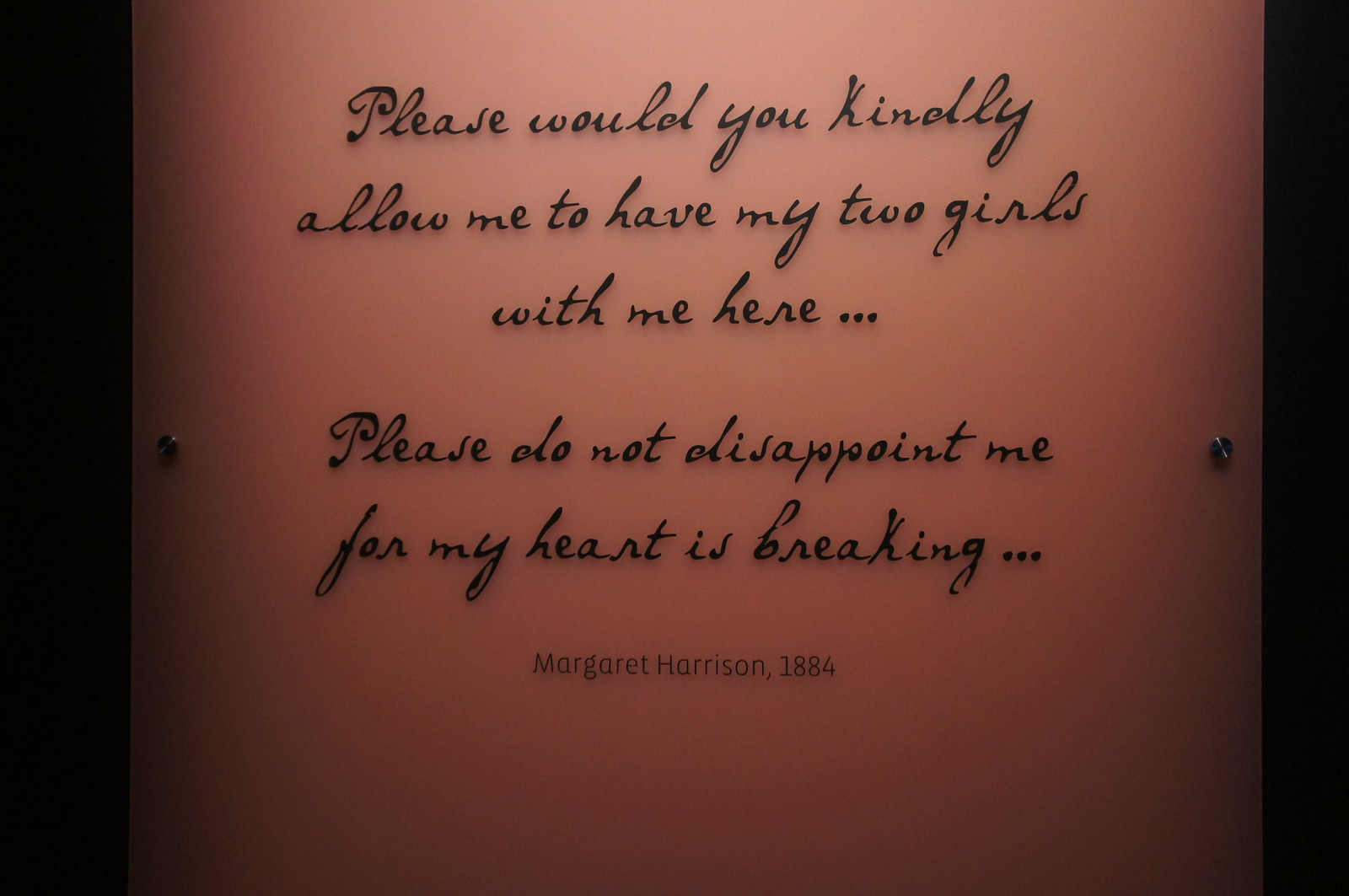The image depicts a photograph of a saying on a light peach-colored background, with heavy shadows cast particularly over the sides and the bottom. The text is written in black cursive at the top, reading, "Please would you kindly allow me to have my two girls with me here... Please do not disappoint me, for my heart is breaking..." Below the cursive text, in a regular and slightly lighter black font, the attribution reads, "Margaret Harrison 1884." The text appears to be meticulously handwritten in ink with precise curves, though it may be a computer-generated cursive style. The saying looks like it has been printed onto a glass or plastic surface mounted on a wall using small silver rivets on both the left and right sides. There are vertical black strips bordering each side of the plaque. The photograph is dark, with only faint illumination from the top, and a subtle drop shadow gives depth to the text against the light background.